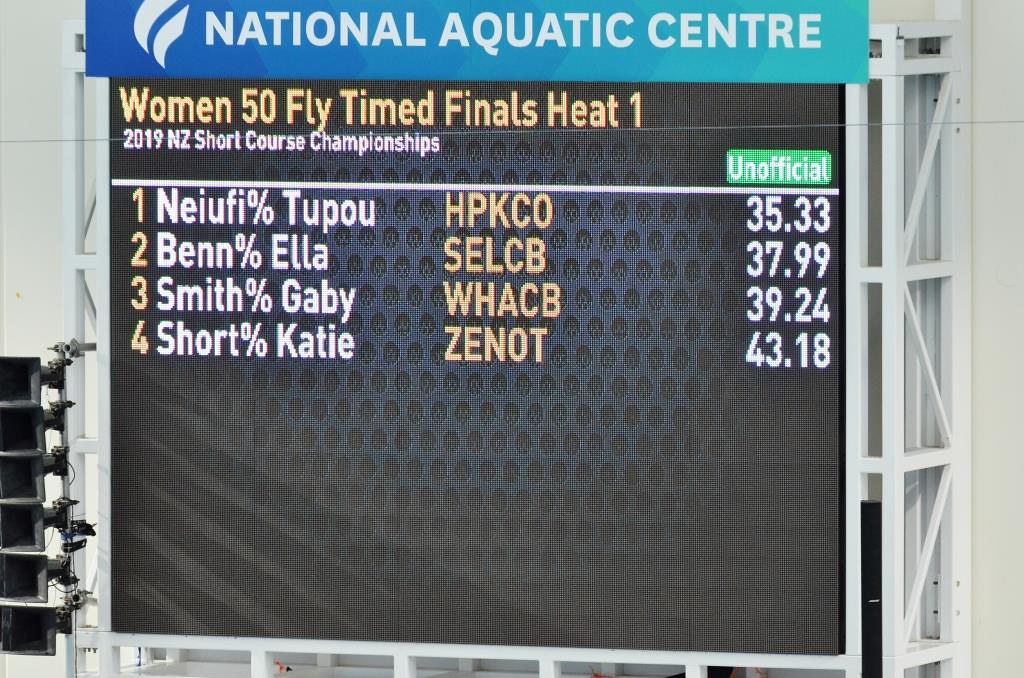The image depicts an electronic scoreboard attached to a white gate at the National Aquatic Center, prominently displayed with a banner in a blue to light green gradient and white text. The scoreboard highlights the results of the Women 50 Fly Timed Finals Heat 1 from the 2019 NZ Short Course Championships, as indicated by the yellow and white headings at the top. There is a horizontal white line segmenting the scores from the headers, with a green rectangle on the far right proclaiming "unofficial" in white text. The details of the timed finals are listed below, with four athletes' names and associations displayed in sequential order. The scores are as follows:

1. Nayufi Topu (HPKCO) - 35.33
2. Ben Ellis (SELCB) - 37.99
3. Smith Gabby (WHACB) - 39.24
4. Short Katie (ZNOT) - 43.18

The overall visual is framed by gray and bordered by parts of a white gate, giving structure to the electronic display, which concludes with a blank section at the bottom.